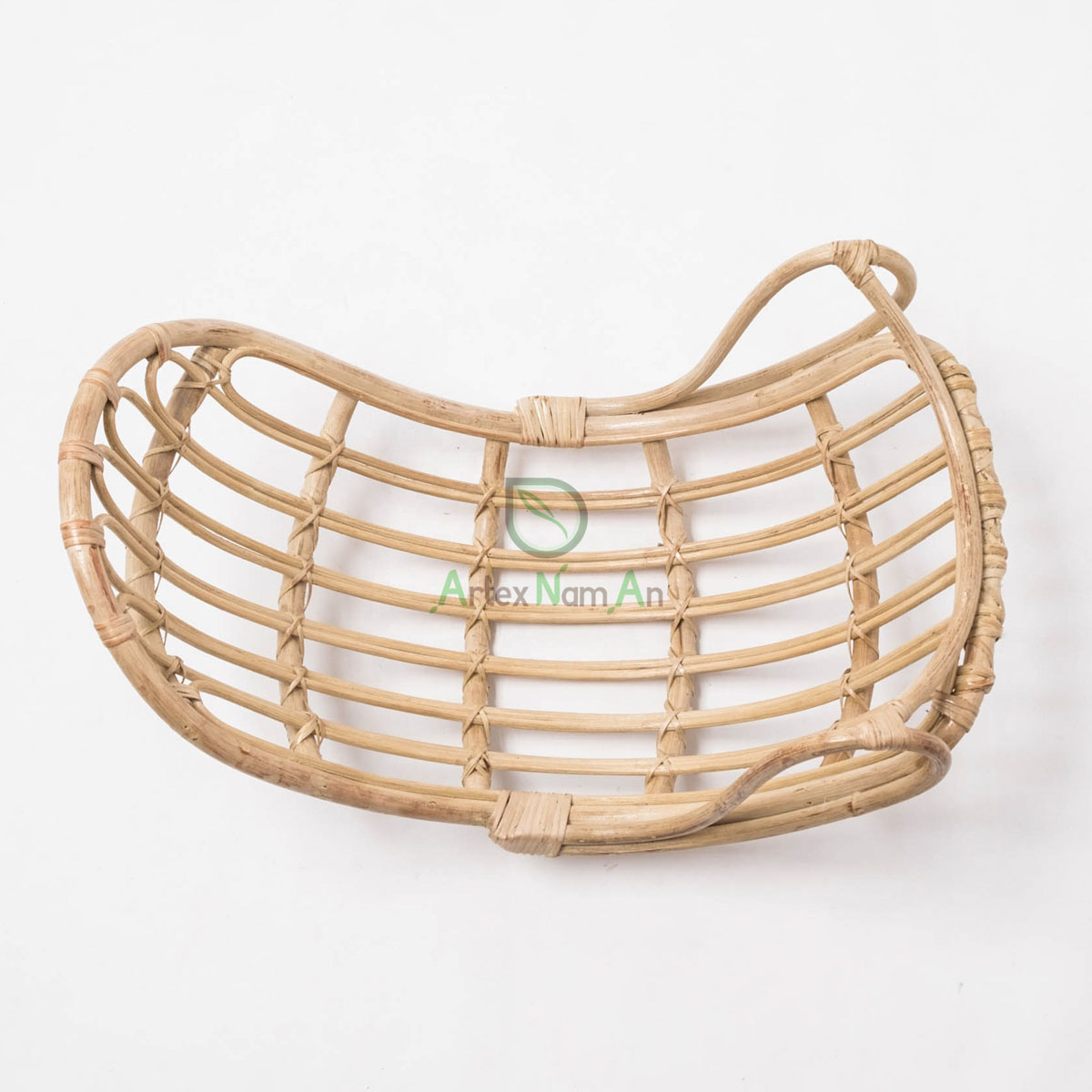The image features a centrally positioned, semi-circular wicker object against a dark gray background. The wicker structure is light brown in color, intricately tied with smaller twine to form its sturdy frame. This artisanal creation resembles a rocking chair designed for back-and-forth movement, cradling the body from head to lower back. It has two lateral handles for grip, aligned laterally with the top facing roughly nine o'clock and the bottom three o'clock. The professional photograph includes a translucent logo in the center, bearing the text "Artex Nom" with the letters A and N highlighted in green and the rest in light gray. The logo features a leaf motif within, adding an artistic touch. The frame of the wicker object is structured almost like a sequence of bow shapes lined together, creating an elegant, wave-like design. Shadows are minimal, enhancing the visibility of the delicate wicker craftsmanship.